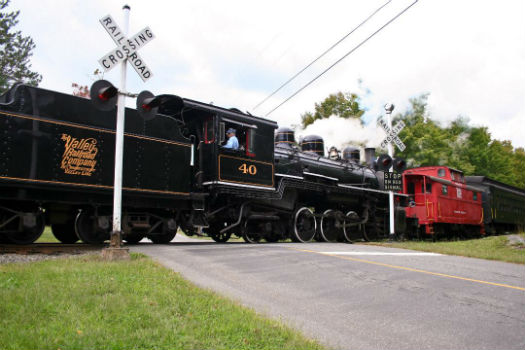This detailed photograph captures a vintage steam-era locomotive crossing a two-lane paved road. The black steam engine, appearing to hail from the industrial age, leads the train with a red caboose immediately following it, an unusual configuration as cabooses typically reside at the train's end. Trailing the red caboose are various black boxcars. The scene unfolds at a railroad crossing marked by two prominent black and white signs, each equipped with red flashing lights. The road, bordered by grass on either side, highlights the nostalgic setting of this old highway crossing as the train moves slowly along its tracks. In the center of the locomotive's visible window, the hint of a conductor can be discerned, adding to the authentic charm of this vintage transportation tableau.